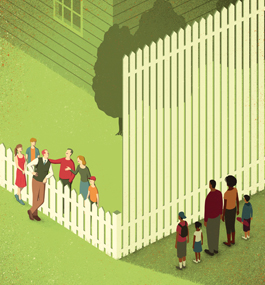In this flat, minimalist cartoon illustration, a white picket fence serves as a powerful symbol of social inequality. The left side of the image depicts a low section of the fence, where a white family stands, easily engaging in conversation with their white neighbor. Behind them, at the top of the image, is a lightly faded house, suggesting the home of the white family. In stark contrast, the right side of the fence is comically tall, almost reaching the top of the illustration, creating a daunting barrier. On this side, a black family stands confined, unable to socialize or see through the towering fence, which casts a shadow over them. This deliberate difference in fence height between the two families highlights the racial divide and underscores themes of racism, social inequality, and exclusion.